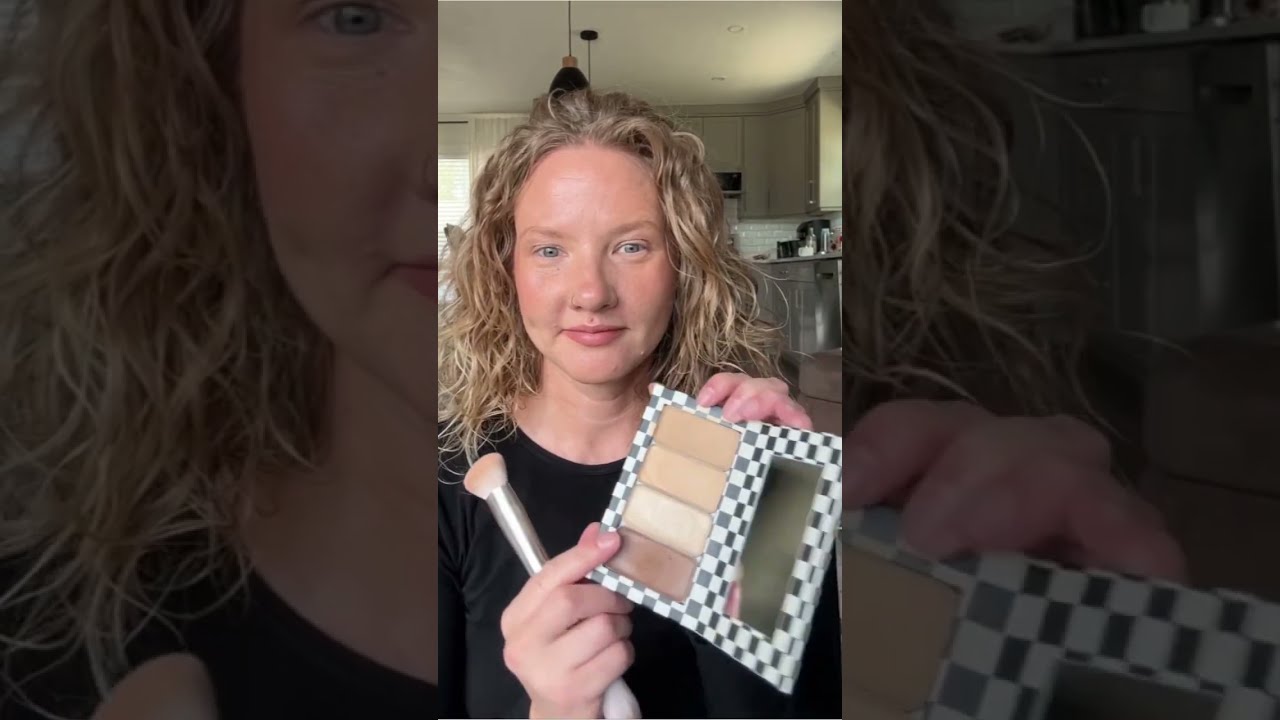The image captures a young Caucasian woman, likely in her teens to 20s, conducting a makeup tutorial, potentially for TikTok or a similar platform. She has shoulder-length, brownish-blonde hair that appears slightly tousled, as if it’s still slightly wet. A light from above illuminates her, and she is standing in what seems to be a kitchen, with cabinets and a refrigerator visible in the background.

The woman is smiling subtly and facing the camera, dressed in a black shirt. She holds a makeup compact in her left hand, displaying various shades of blush or skin-tone makeup. The compact features a checkered black and white pattern around its border, with four shades on the left and three on the right side of the open makeup tray, accompanied by a mirror. In her right hand, she holds a long, silver makeup brush. Her facial features include blue eyes, light blonde eyebrows, and light red lips. The right and left thirds of the image appear to be zoomed-in, semi-bright sections, focusing on the compact in one hand and the makeup brush in the other, respectively. The woman seems to be demonstrating how to apply or blend makeup on her face.